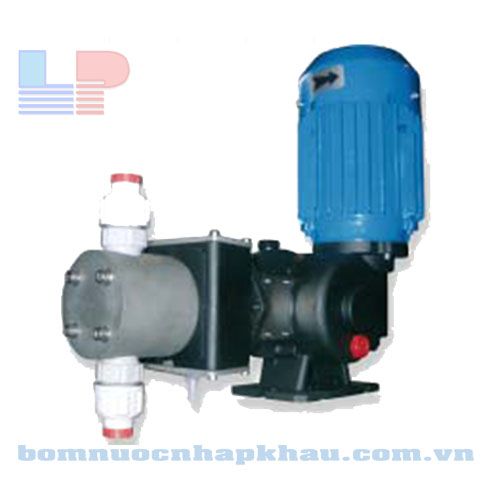This detailed image showcases a mechanical device, likely a water filtration or pumping mechanism, set against a clean white background. The device features a large, cylindrical blue component with vertical texturized gripping and an arrow pointing to the right. Most of its body is black, incorporating a red button. Adjacent to the blue section, there's a gray cylinder extending outward, with two white dispensers at the bottom, each capped in red. In the upper left corner, the letters 'LP' are displayed with 'L' in blue and 'P' in a red or pink hue, accompanied by five lines under each letter. A website, "bomnuocnhapkhau.com.vn," is faintly visible at the bottom, potentially hinting at Vietnamese origins or market. The colors present in the image include blue, red, white, gray, and black. This configuration suggests the image might be part of an advertisement or educational material promoting the device.